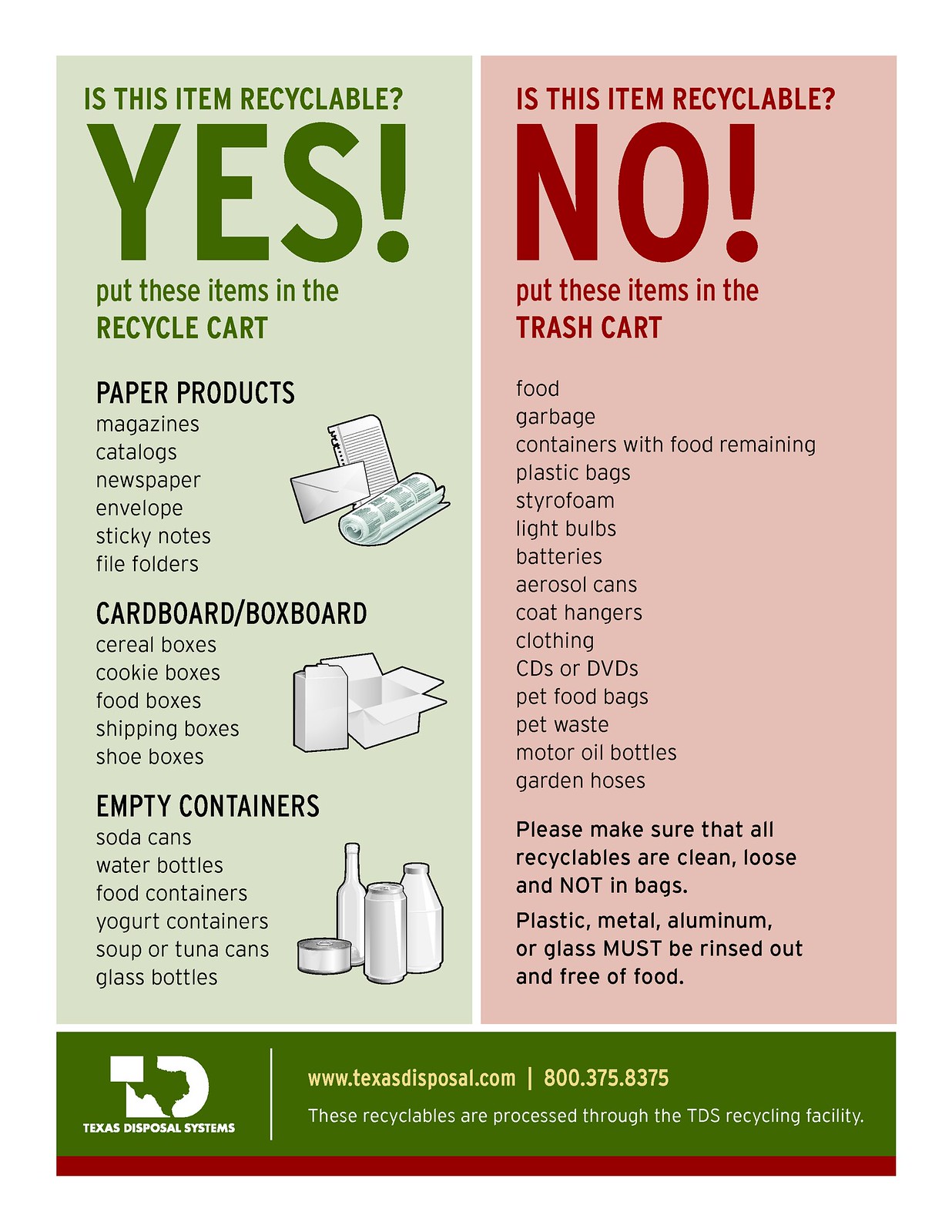This rectangular advertisement from Texas Disposal Systems provides comprehensive recycling instructions, partitioned into two color-coded sections. The left section, colored green, is titled "Is this item recyclable? Yes, put these items in the recycle cart" and lists recyclable materials with accompanying images, including paper products such as magazines, catalogs, newspapers, envelopes, sticky notes, file folders; cardboard and box boards; and empty containers like soda cans, water bottles, yogurt containers, and glass bottles. The red-colored right section, titled "Is this item recyclable? No, put these items in the trash cart" lists non-recyclable items such as food, garbage, containers with food remaining, plastic bags, styrofoam, light bulbs, batteries, aerosol cans, coat hangers, clothing, CDs, DVDs, pet food bags, pet waste, motor oil bottles, and garden hoses. The bottom of the advertisement features a solid green banner with additional instructions— "Please make sure that all recyclables are clean, loose, and not in bags. Plastic, metal, aluminum, or glass must be rinsed out and free of food."— along with the Texas Disposal Systems logo, their website www.texasdisposal.com, and contact number 800-375-8375, emphasizing that these recyclables are processed through the TDS Recycling Facility.